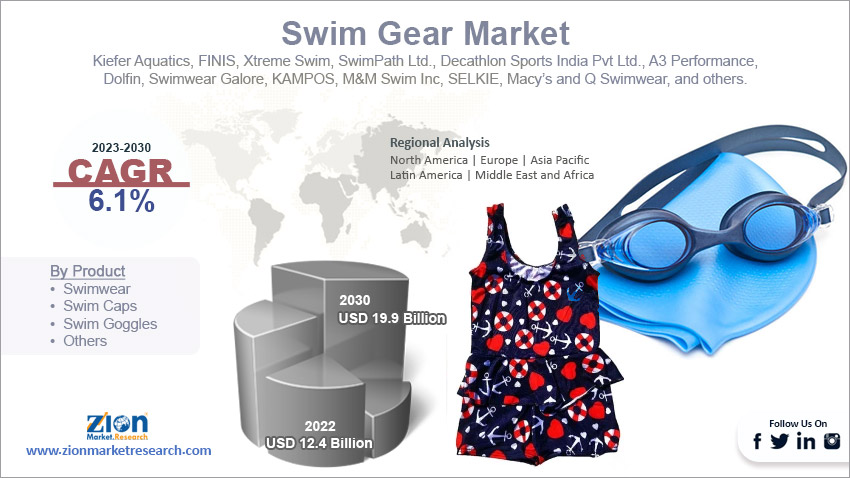The infographic titled "Swim Gear Market" features a detailed analysis of the swimwear industry from 2023 to 2030. It includes a list of prominent swimwear brands such as Kiefer Aquatics, Finis, Extreme Swim, Swimpath Ltd, Decathlon Sports India Private Limited, A3 Performance, Dolphins, Swimwear Galore, Campos, M&M Swim Incorporated, Selke, Macy's, and Q's Swimwear. The infographic is bordered by a thin dark bluish-gray line and has a white background with dark bluish-gray text.

Prominently displayed on the left is a key statistic indicating a Compound Annual Growth Rate (CAGR) of 6.1%. Below this is a regional analysis covering North America, Europe, Asia-Pacific, Latin America, the Middle East, and Africa, complete with a world map shading the continents in various shades of gray. On the bottom of the infographic is a hybrid pie and bar chart revealing revenue projections: $19.9 billion USD for 2030 and $12.4 billion USD for 2022.

In the middle right, there is an image of swim gear, including a swim cap and goggles, while to the bottom middle, there is a girl’s bathing suit adorned with life rafts, anchors, and hearts. The colors used throughout the infographic range from light blue, darker blue, red, navy blue, gray, white, to light gray. Zion Market Research is credited with the infographic's data and analysis.